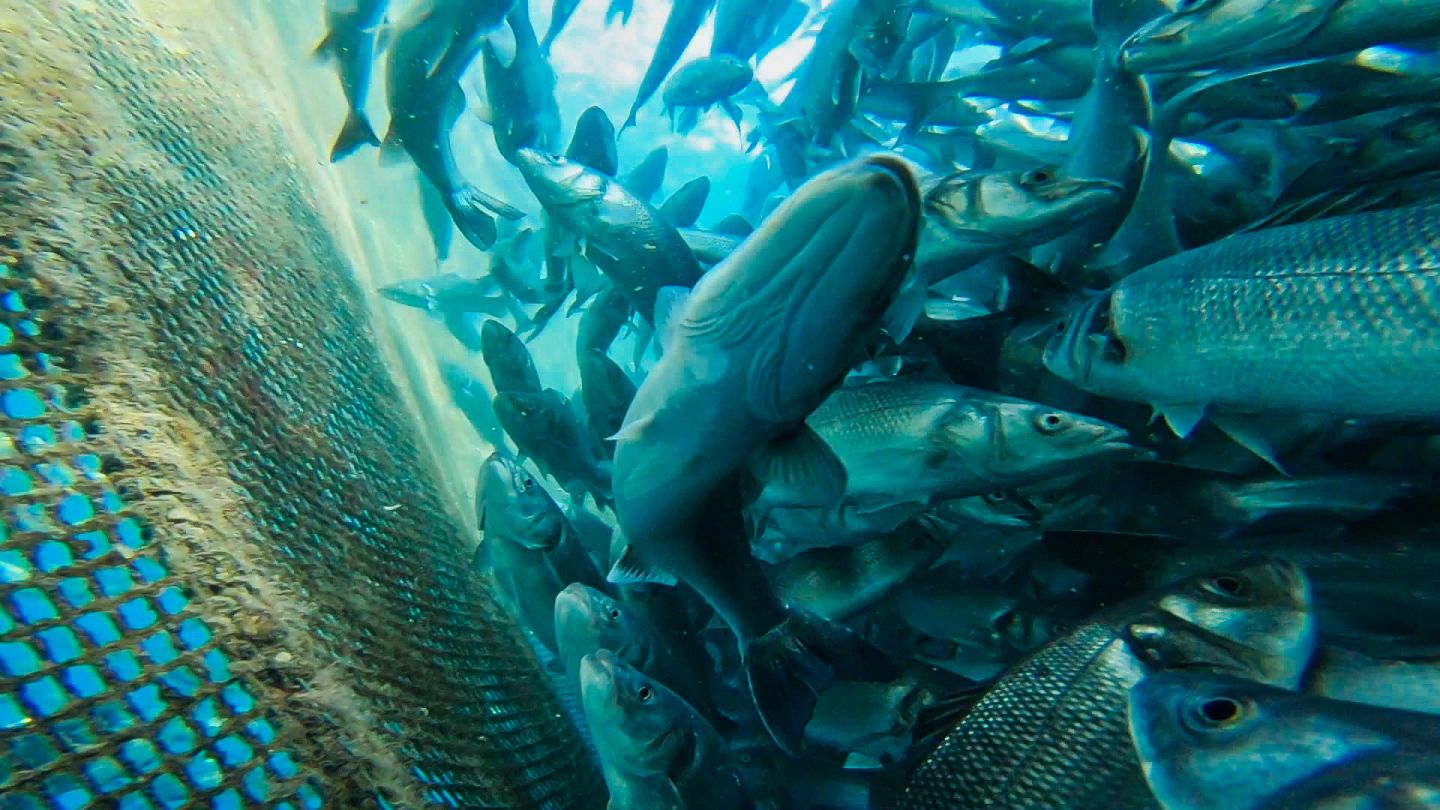This underwater photograph captures a dense school of long, slender fish, silver-scaled with somewhat buggy eyes, all cramped together and swimming in various directions under the blue water. The image shows sunlight filtering through the water surface, casting a blue hue over the scene. On the left side, a large, commercial fishing net is visible, made of sisal or a similar brown rope. The net appears almost like a giant sisal rug capturing the fish, except for the leftmost edge where the mesh is loose enough to see the clear blue water through it. The net is coated with algae, dirt, and moss, indicating years of use, contributing to the overall color palette of silvers, blues, grays, browns, and tans.